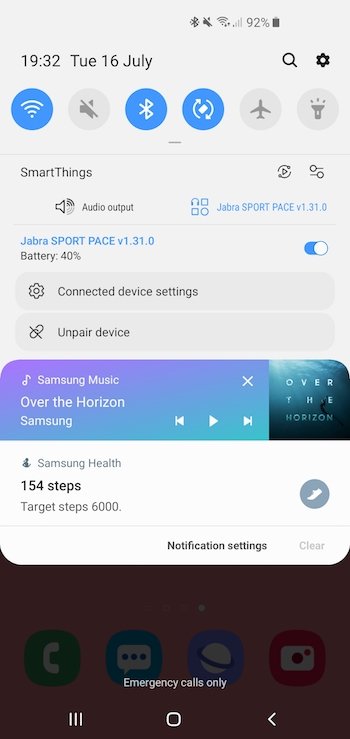The image is a screenshot from a smartphone. The top section of the screenshot has a light gray background, displaying essential status icons, including Wi-Fi, muted speaker, Bluetooth, refresh, airplane mode, and a flashlight. The top bar also shows the time, 19:32, and the date, Tuesday, 16 July.

Below this bar, a pop-up box occupies the middle to bottom part of the screen, partially muting the background. At the top of this box, it says "SmartThings," followed by "Audio output," and then lists "Jabra SportPace V1.31.0," with a battery indicator showing it at 40%. To the right of this information, there is a slider indicating that the device is turned on.

Further down, a gear icon appears next to the text "Connected device settings." Below this, a Bluetooth icon with the text "Unpaired device" can be seen. Continuing downward, the interface shows "Samsung Music" with the title "Over the Horizon," along with controls for playing, rewinding, and forwarding the track. Lastly, a fitness tracker display notes "154 steps," with a target of "6,000 steps."